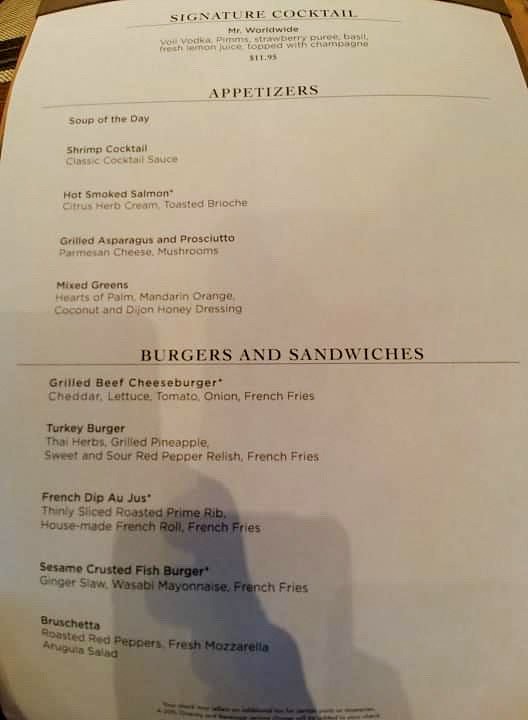A close-up photograph of a restaurant menu is presented, resting on what appears to be a table. The table's edges are dimly visible at the very top left and right, suggesting a subtle presence of a tablecloth. The menu itself is printed on a simple white sheet of paper with black text. It is organized into three distinct sections: "Signature Cocktail," "Appetizers," and "Burgers and Sandwiches."

A notable feature of the image is the shadow cast upon the menu. Both a lighter and a darker shadow are visible, likely from the person taking the photograph. The outline of a hand, arm, and the phone used to capture the image can be discerned within this shadow.

The "Signature Cocktail" section highlights a single item named "Mr. Worldwide," priced at $11.95. The "Appetizers" section lists several dishes, including Soup of the Day, Shrimp Cocktail, Hot Smoked Salmon, Grilled Asparagus and Prosciutto, and Mixed Greens; however, specific prices for these items are not provided. The "Burgers and Sandwiches" section offers five choices: Grilled Beef Cheeseburger, Turkey Burger, French Dip au Jus, Sesame Crusted Fish Burger, and Bruschetta. The bottom of the menu contains some fine print, but it is too small and indistinct to be read clearly.